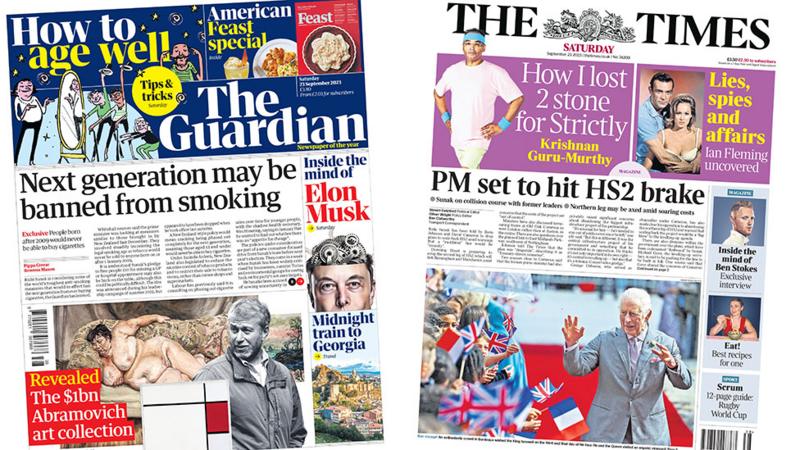This image features the front covers of two magazines. The first magazine showcases a series of noteworthy headlines and visuals:

- At the top, a prominent blue box reads "How to Age Well." 
- A small yellow circle provides tips and tricks.
- In the top-right corner, a square announces an "American Feast Special."
- A little red book titled "Feast" is also highlighted.
- The cover displays pictures of people enjoying themselves in front of a large mirror.
- The magazine's title, "The Guardian," is written in bold white letters.
- Key articles include "Next Generation May Be Banned From Smoking" and "Inside the Mind of Elon Musk," which is accompanied by an illustration of Musk with intricate cogs and gears within his brain.
- Other notable mentions are "Midnight Train to Georgia" and the revealing of the "Sibbin Abramovich Art Collection," featuring an image of a voluptuous, naked woman reclining on a sofa.
- Also present is a white square with black lines and a red box containing a man's picture.

The second magazine, titled "The Times," includes:

- A central image of dragons.
- Headlines such as "Saturday: How I Lost Two Stone for Strictly" by Krishnam Guru Murthley, with a picture of a man dressed in white featuring blue accessories.
- A purple headline that reads "Lies, Spies, and Affairs – Fleming Uncovered."
- "PM Set to Hit HS2 Break."
- A large image that appears to be of Prince Charles.
- On the right side, there are smaller images and texts, including "Inside the Mind of Ben Stokes," "Eat," and "Scream" at the bottom.